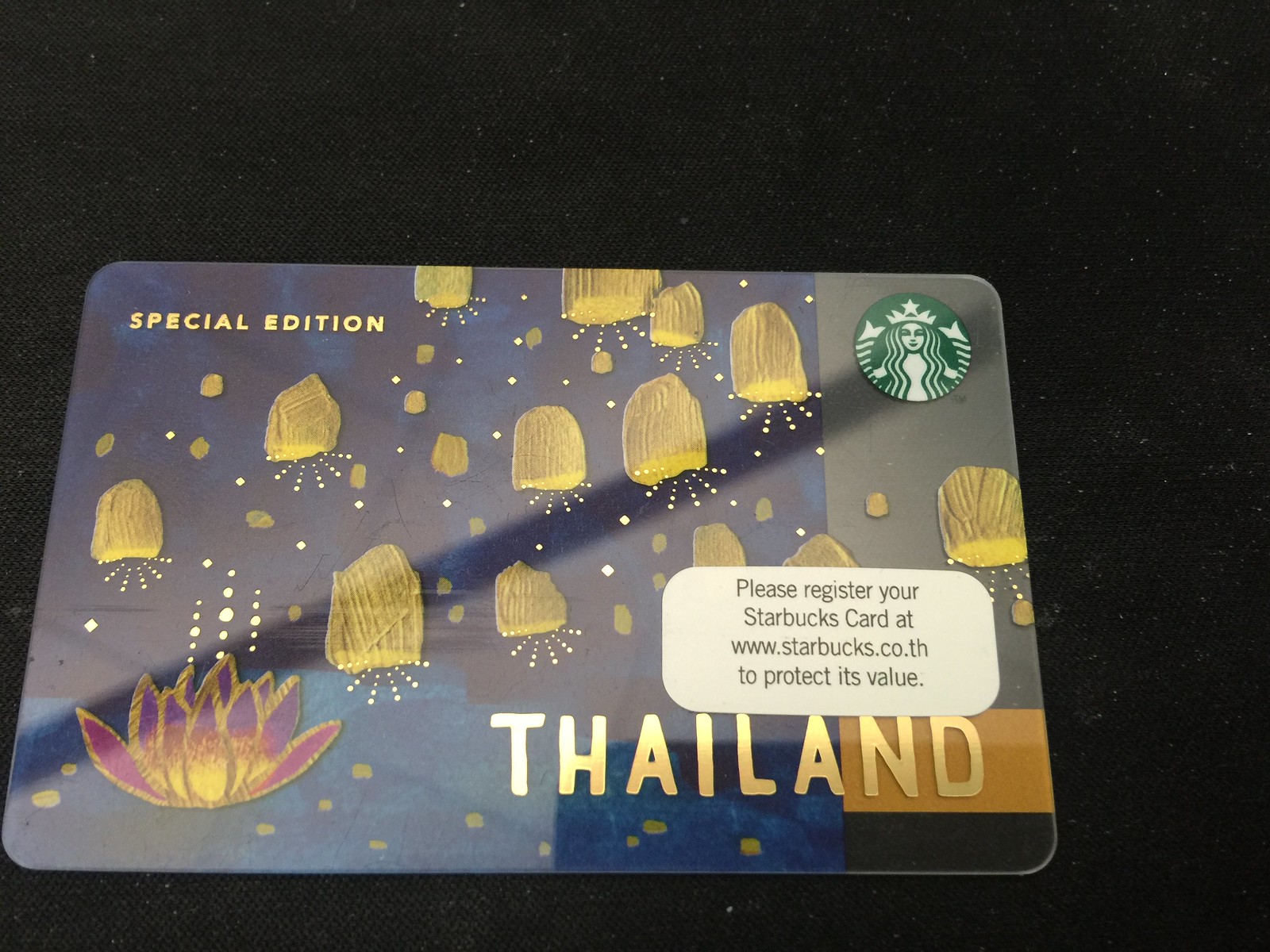The photograph features a Special Edition Starbucks gift card prominently positioned on a black surface, which could be fabric or a tabletop. The card itself is rich in detail and vibrant colors, ranging from dark blue to black, yellow, green, pink, purple, and orange. In the top left corner, it bears the label "Special Edition," while the iconic green Starbucks logo is situated in the top right corner. The bottom right corner of the card reads "Thailand" in gold lettering, with a prompt above it to register the card at www.starbucks.co.th to protect its value.

The design on the card includes a series of paper lanterns or possibly jellyfish-like figures floating upward, each emitting rays of light depicted as dotted lines. These lanterns have six rows of dots extending from them. Additionally, there is an image of a flower floating in water located at the bottom left of the card, also releasing light beams in the form of three rows of dots. The overall image is clear, well-lit, and captures all intricate details of the card effectively.